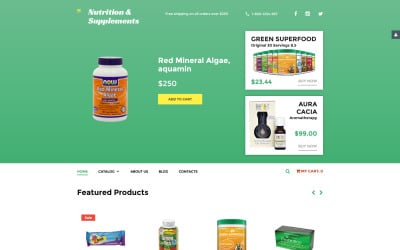The homepage appears to represent an online store specializing in supplements and nutrition products, with a distinctly bohemian or alternative wellness vibe. The top of the page showcases a prominent product against a green background: a jar labeled "Red Mineral Algae, Aquamin," priced at $250. Additional text mentions "Green Superfood" or "Acacia."

Below this featured product section, there are four images representing other items, though these lack descriptive text. The layout and design of the website come across as somewhat poorly executed, lending an impression of being inexpensive and potentially untrustworthy. With high-priced items displayed on a seemingly low-quality site, it evokes a sense of a dubious market, reminiscent of under-the-table or black market transactions. Overall, the website conveys a peculiar and suspect appearance.